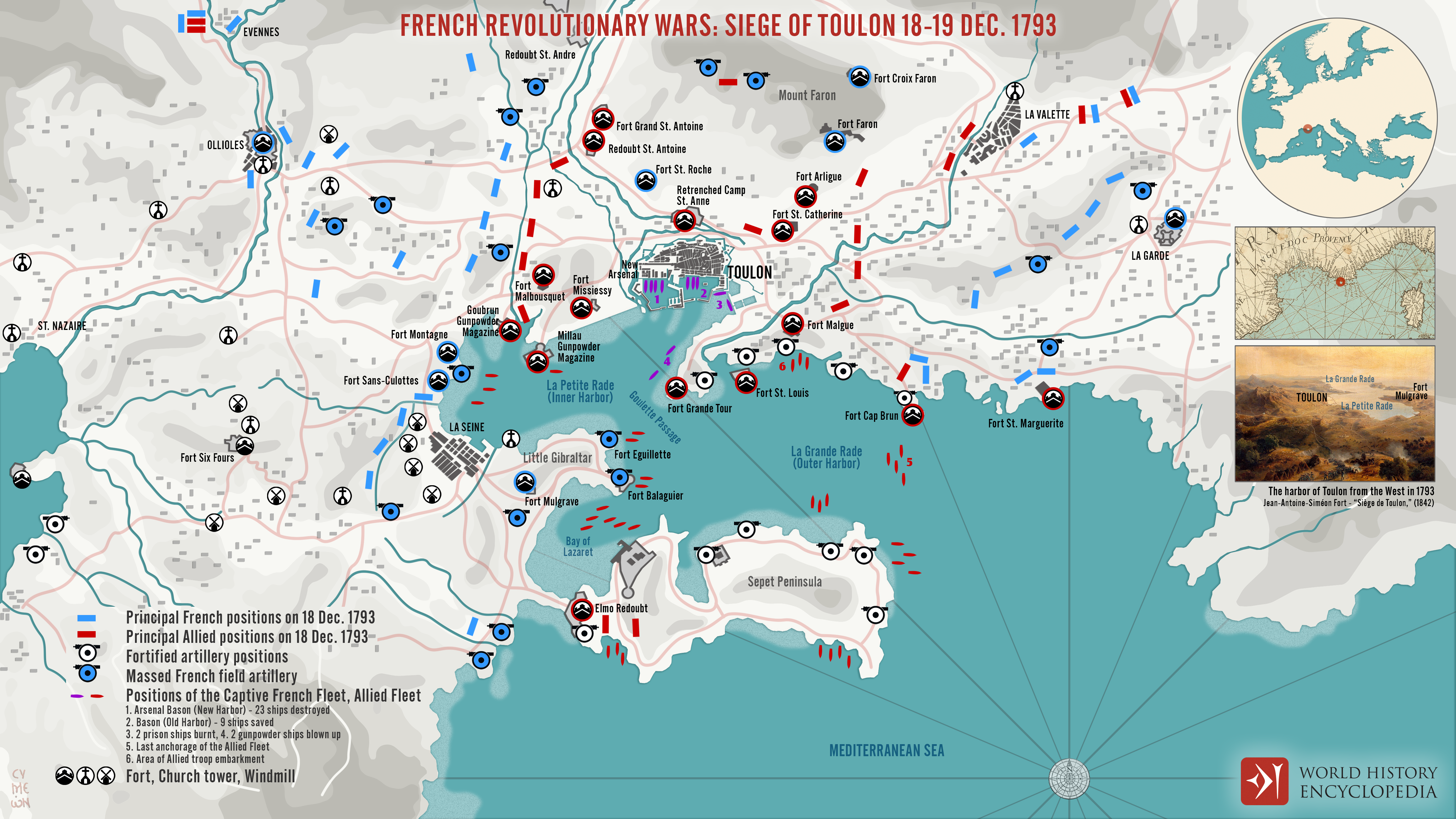This detailed map illustration, titled "French Revolutionary Wars: Siege of Toulon, 18-19 December 1793," features a central, prominently labeled depiction of a European region during a pivotal historical moment. The map uses various color codes and symbols to indicate different strategic positions: light blue lines for principal French positions on December 18, 1793, red lines for principal Allied positions on the same date, white cannons for fortified artillery positions, and blue cannons for massed French field artillery. 

The map is supplemented by a key located in the bottom left corner, explaining these symbols in detail. The landscape-oriented map primarily displays white landmasses with turquoise-colored sections representing the Mediterranean Sea. Roads and other significant routes are highlighted in blue, yellow, and pink, providing a comprehensive overview of the battlefield layout.

A circular icon on the top right shows a small globe, pinpointing the specific region depicted in the larger map. Underneath are two additional landscape illustrations: the top one providing an outer regional view and the lower one offering a detailed landscape perspective with accompanying text. The image is further endorsed by a red square logo and "World History Encyclopedia" credit at the bottom right corner, reinforcing its educational purpose. This detailed, colorful map art effectively captures the historical significance and strategic intricacies of the Siege of Toulon during the French Revolutionary Wars.